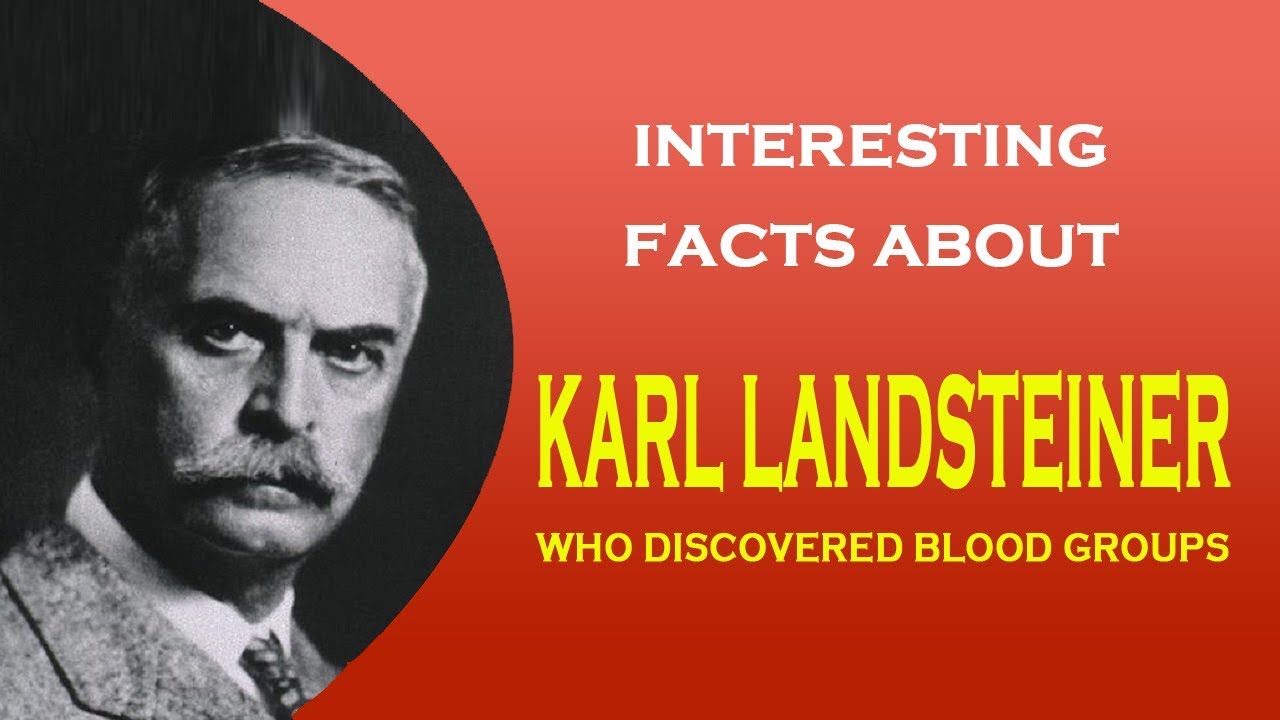The image appears to be a carefully designed educational piece, possibly for a book or a science exhibit, and could also function as a slide in a PowerPoint presentation. It prominently features a stern black-and-white portrait of Carl Landsteiner on the left. Landsteiner, identified as the man who discovered blood groups, has short hair, dark eyes, and a full, bushy mustache. He is dressed in a suit with a white shirt and a tie, and his expression is serious and intent.

This portrait is set within a curved, half-circle design that takes up about a third of the image. The remainder of the background, which transitions from a lighter whitish red at the top to a darker red at the bottom, features text. At the top, in white font, it reads "interesting facts about," while below that, in larger yellow font, it states, "Carl Landsteiner who discovered blood groups." The text and layout suggest the image could serve multiple educational purposes, providing a visually impactful introduction to Landsteiner's contributions to science.